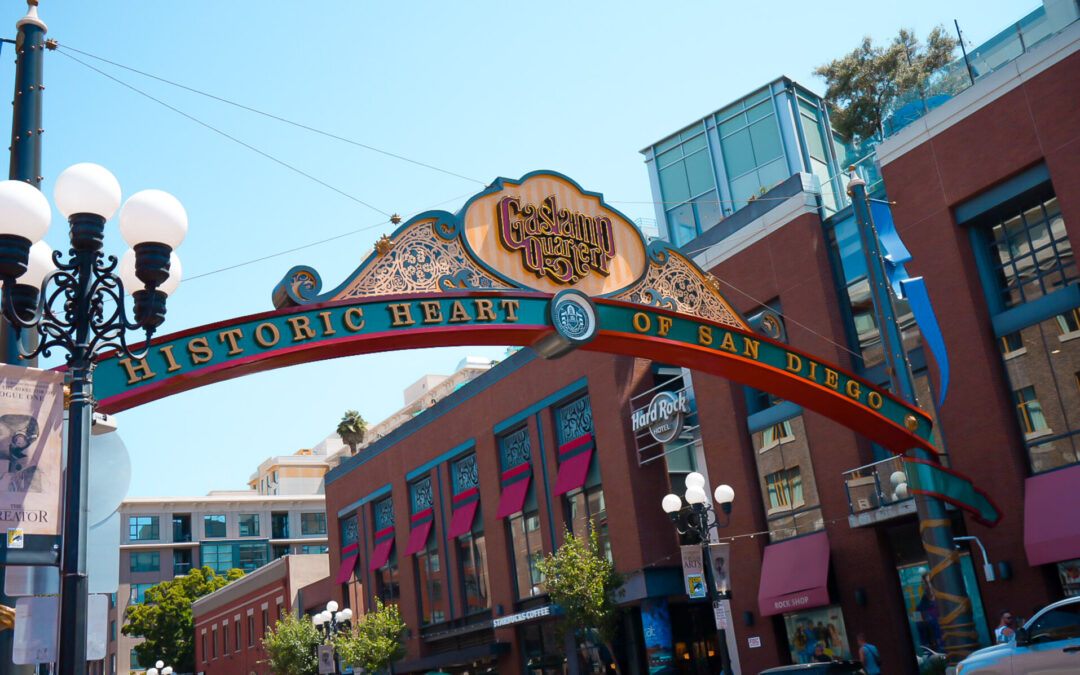The image captures a sunny day with a clear, light blue sky in the heart of San Diego. Dominating the scene is a beautifully ornate, arching sign that reads "HISTORIC HEART OF SAN DIEGO" in large, gold capital letters. This sign is set against a blue background with red trim along the arch. At the center of the archway, within a fluted wooden cutout with a blue outline, there's a badge that reads "Gaslamp Quarter" in purple letters on a pink and white striped background. Supporting the arch are two blue metal poles adorned with blue banners. To the left, there is an old-style street lamp with five white bulbs. Nearby, a brick building with colorful window treatments and red awnings houses a Hard Rock Café, its sign clearly visible. More buildings, characterized by glass and brick, extend into the background. Cars and people are visible on the street below, adding to the lively urban scene.